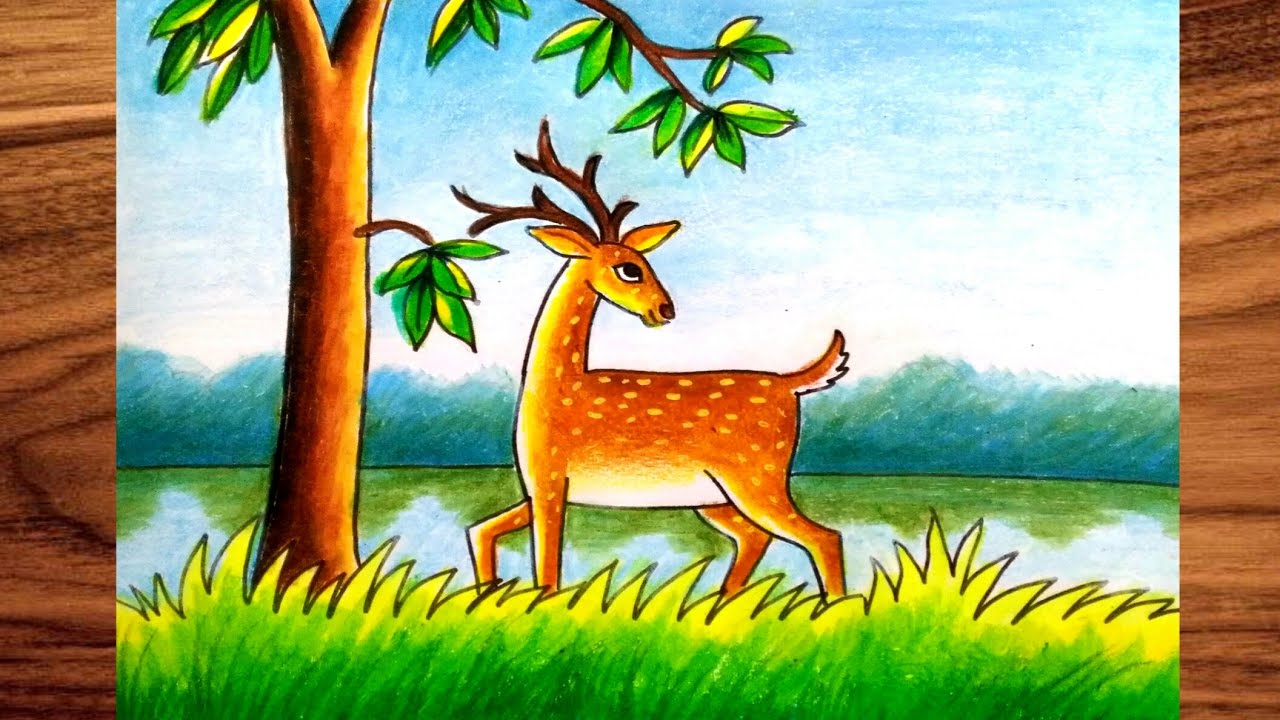This color illustration, rendered in crayon and markers, depicts a stylized yet representational deer positioned centrally in a landscape scene. The deer, with a light golden honey coat adorned with elliptical white spots and a white underbelly, stands in profile, facing left while its head is turned back to the right displaying a pleasant expression. The deer’s dark brown antlers curve gracefully above its head, and its yellowish-brown ears frame black pupils set in white eyes above a darker snout.

In the foreground, vibrant green grass with lighter yellow tips outlined in black stretches across the bottom of the image. Behind the deer, a tranquil blue lake reflects shadows of dark green mountains that rise on the horizon. The sky above is a soft blue, interrupted occasionally by white clouds and a tree line composed of dark green foliage.

To the left of the deer, a dark brown tree trunk extends upward, forming a V shape with small and larger branches adorned with green leaves. The overall composition sits on a finished wooden table characterized by a lighter wood tone contrasted with thick, dark grain patterns. The illustration, rendered with a sense of animated realism, evokes a serene outdoor scene with its rich, detailed textures and colors.